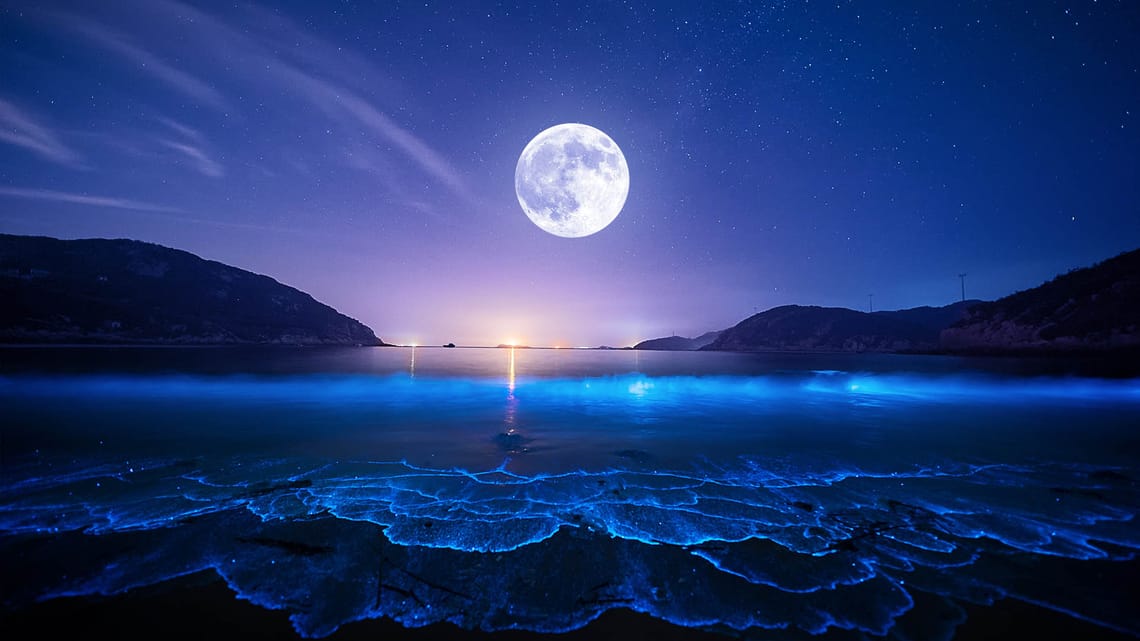This nighttime photograph captures a captivating coastal scene under a strikingly large full moon. The scene is framed by shorelines that extend into the flat, dark waters stretching to the horizon, where the faint outline of an island can be glimpsed in the distance. The bottom of the image features waves from the ocean or lake rushing ashore, with the water reflecting an ethereal blue glow, perhaps illuminated by bioluminescent organisms. This glow is most vivid in the central wave crashing onto the beach. Across the water, a series of mysterious lights can be seen, possibly from distant boats, adding intrigue to the landscape.

The sky presents a gradient of colors, transitioning from lighter purples near the horizon to deeper blues towards the upper corners. A few streaky white clouds drift in the top left portion of the sky. The most arresting feature, however, is the massive full moon, so large and detailed with gray craters that it seems almost surreal, dominating the dark, navy-shaded heavens. Its light not only illuminates the water but also creates a reflective path across the surface, enhancing the tranquil yet otherworldly ambiance. Scattered across the sky are white specks of stars, completing this enchanting nocturnal vista.